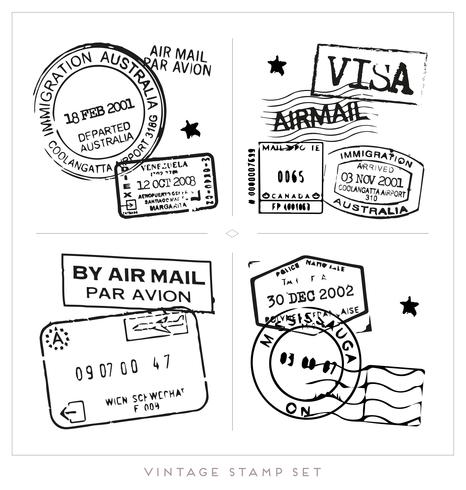This black and white image features a collection of vintage stamps, arranged in a square and resembling a postcard or a sticker set. Each of the four stamps showcases different text and dates, giving it a cohesive yet diverse appearance that would appeal to a vintage stamp collector. The top left stamp reads "Air Mail Par Avion, Immigration Australia," dated October 12, 2008, while the top right stamp says "Visa Air Mail" and is dated November 3, 2001. In the lower left corner, the stamp features the text "Buy Air Mail Par Avion" along with a number, 09070047. The lower right stamp is marked with the date December 30, 2002, and includes a star graphic. The overall design and arrangement, along with the monochromatic color scheme, give it a nostalgic feel reminiscent of historical postal artifacts.